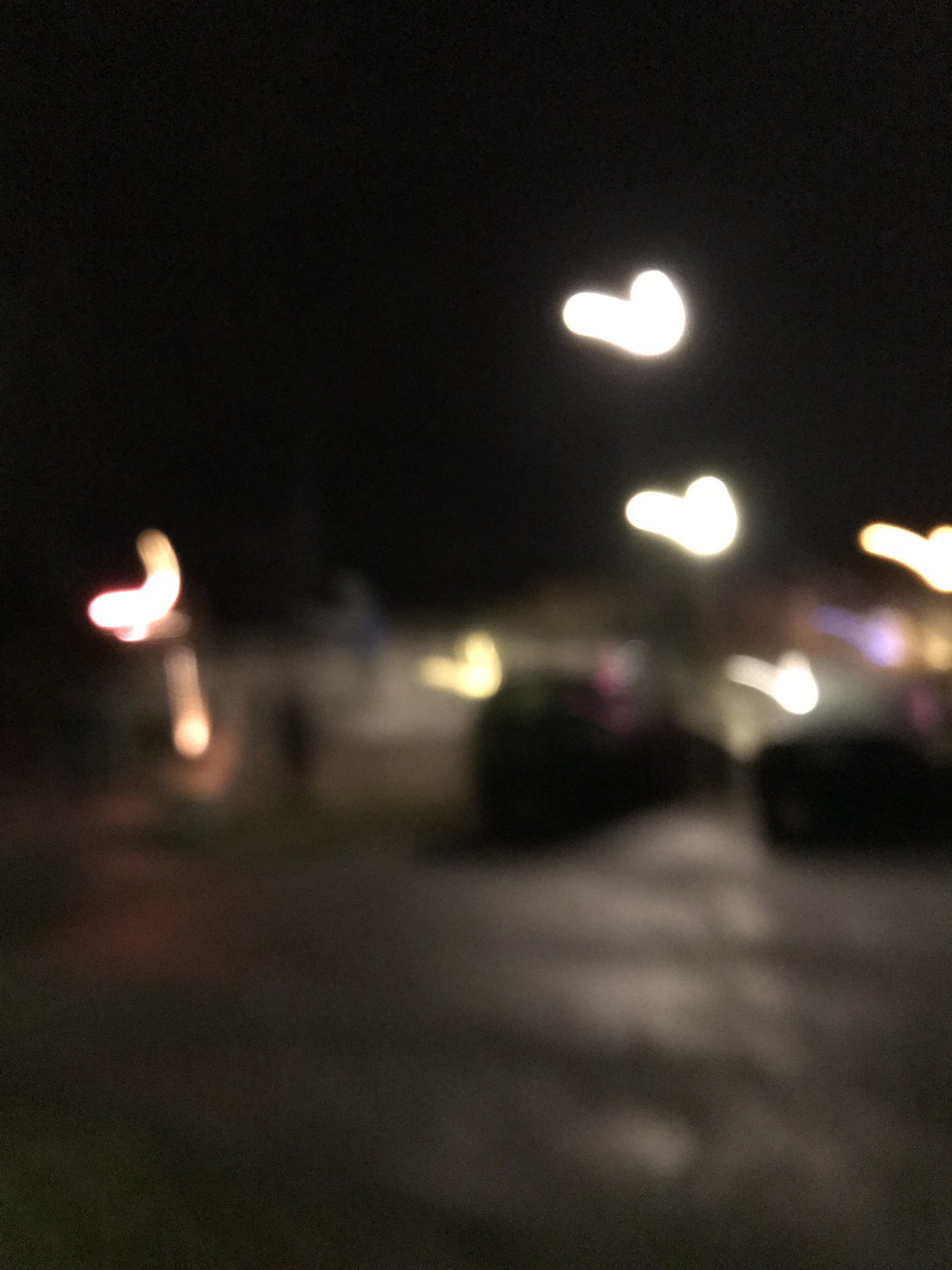The image is an extremely blurry and dark night-time scene, capturing what appears to be a parking lot or a street with elements of both a residential and urban setting. Central to the image are two dark-outlined cars parked towards the right side. The surrounding area, rendered in dark gray, is punctuated by indistinct white structures that could be houses or buildings; one such building extends from the left to the right side, seemingly containing a door. At the top of the image, the night sky is black and featureless save for about seven glowing lights, which are scattered and appear as floating, blurry orbs arranged in a vague slanted V-shape. Some of these lights have a unique appearance, such as one resembling a 'C' on top of a stick. The overall lack of clarity suggests the photo was taken in motion or in poor lighting conditions.